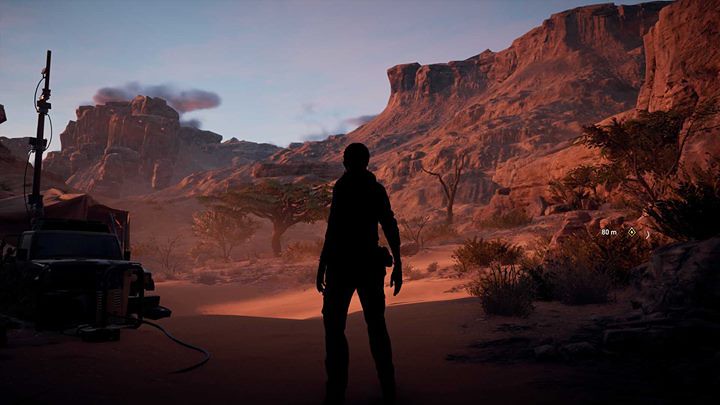A detailed caption for the described image might be:

"In this landscape-oriented screenshot from a third-person perspective video game, the scene is set against a dusky, orange-tinged desert backdrop. The main character, seen from behind and silhouetted against the fading light, stands as a dark figure amidst the expansive surroundings. In the distance, tall red rock canyons rise majestically, their rugged forms partially obscured by dust. Adding to the immersive gameplay experience, a waypoint marker appears on the right side of the screen, indicating '80 meters' with an arrow, guiding the player's next move. The setting sun casts a golden hue, painting the scene with the warm glow of the golden hour, enhancing the dramatic and captivating atmosphere."